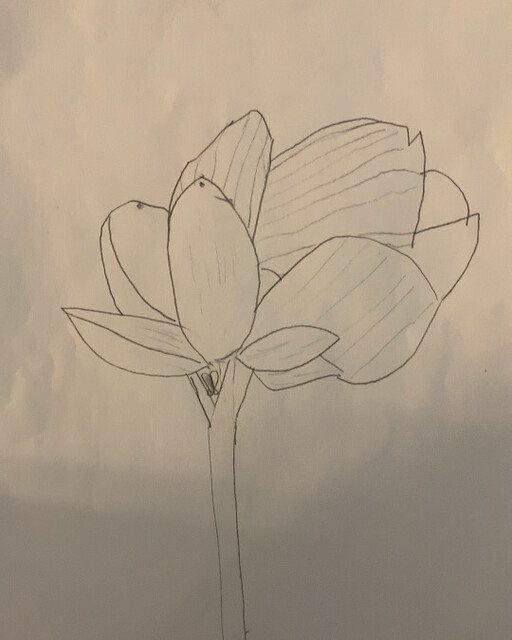This is a detailed pencil drawing of a flower, possibly an orchid, set against a wrinkled white piece of paper, likely standard printer, graphing, or drawing paper. The paper has noticeable creases in various parts, including the top, left, bottom right, and top right corners, with shadows along the bottom of the page. 

The flower's delicate structure begins with a slender stem originating from the bottom center of the page. This stem branches off into a slight V shape and is flanked by multiple petals and leaves. The petals display a mix of shapes—some are ovular and pointed at the tip, while others are wider, unorthodox, and blob-like. A section of the flower features oblong leaves, with one leaf standing upright, a second leaf marked with a line, and another more pointed leaf emerging from the bottom. As the stem curves to the right, it reveals more irregularly shaped, striped leaves.

The petals vary in their detailing, with some exhibiting numerous vertical and horizontal striations, and others adorned with just a few lines. The flower itself dominates the center of the page, showcasing intricate detailing synonymous with meticulous pencil work.